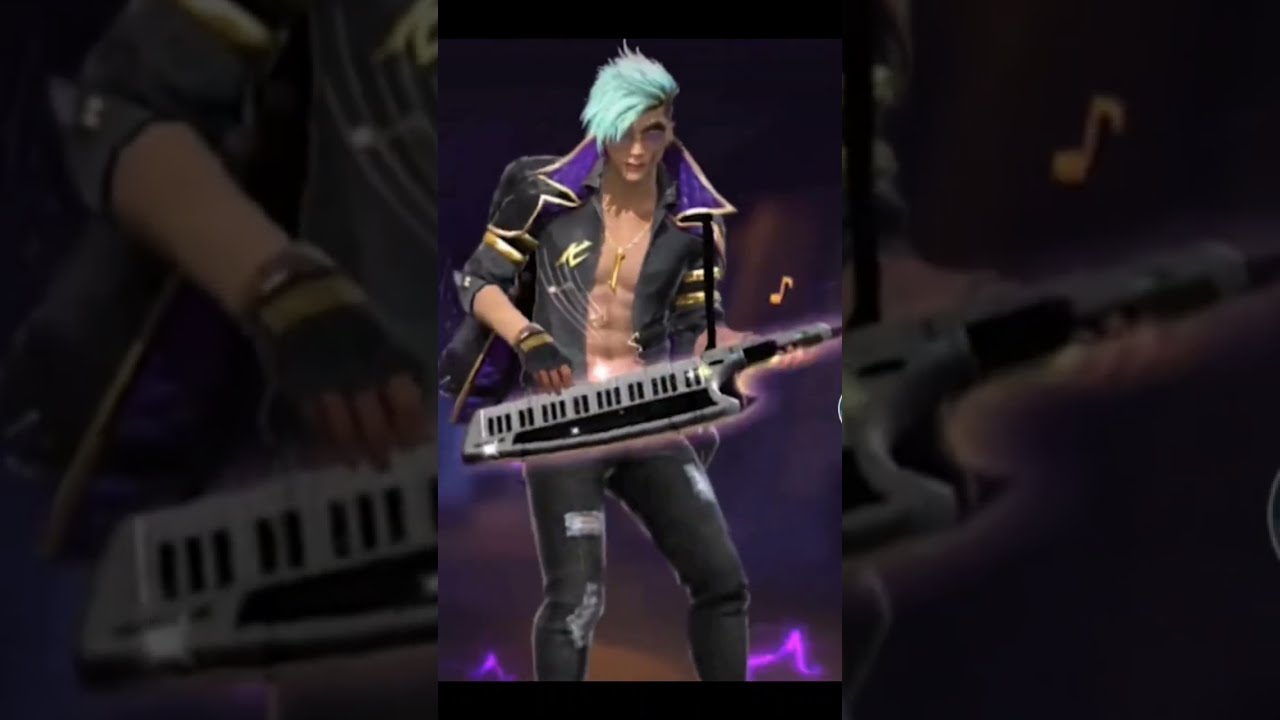The image is a horizontally rectangular box divided into three sections: a dark, out-of-focus left section showcasing a man's right arm touching a keyboard; a well-lit, detailed middle section featuring a rock star playing a keyboard guitar with his right hand while his left hand holds the neck, his light blue, emo-styled hair partly covering his right eye. He wears an open leather vest or black jacket with yellow embellishments and a wide, pointed purple collar, along with black jeans marked with patches. The background is a purplish hue. The right section focuses on the end of the keyboard and is somewhat dark and blurry, showing the man's arm supporting the instrument and featuring a yellow musical note above it. A faded, zoomed-in overlay of the same image serves as the background, adding a layered, almost transparent effect to the overall graphic.